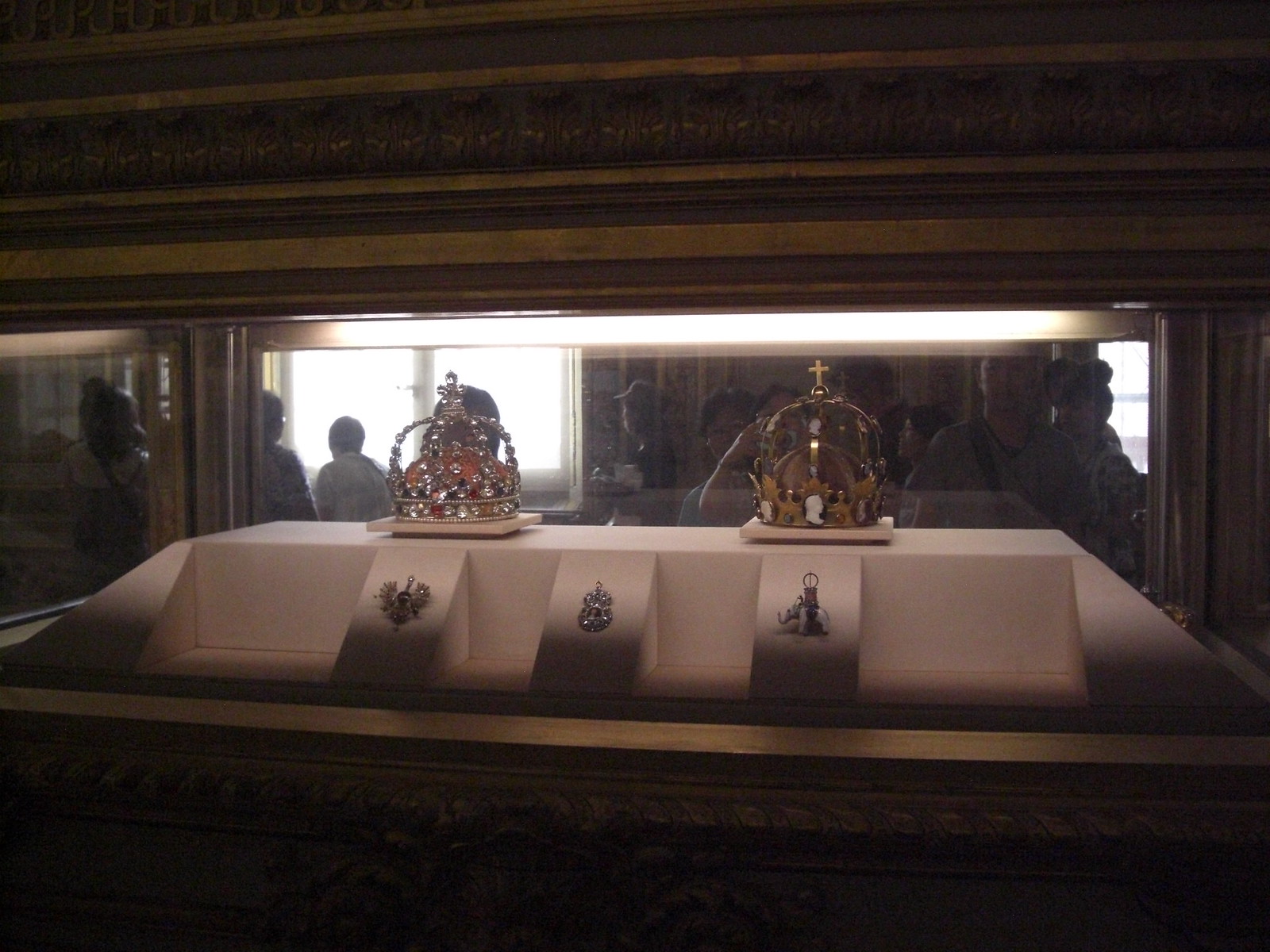This photograph, taken in the dim, ambient light of the Louvre Museum in Paris, captures a beautifully ornate display case housing two magnificent crowns. The case is constructed of glass with brass and stainless steel trim, and features carved wood with gilded accents that lend it an air of royal opulence. Inside, the crowns are prominently showcased on a raised platform, each spotlighted by subtle overhead lighting. The crown on the left is encrusted with what appears to be diamond and coral-colored elements, while the crown on the right, adorned with gold and possibly ivory, is topped with a small cross. The right crown also features a royal eagle motif.

Beneath the crowns, the display extends downward with three angled shelves adorned with various jewels, brooches, and detailed diagrams. The foreground of the photograph captures the glass case entirely enclosed, framing the scene elegantly.

In the background, reflections and possibly the other side of the display show museum visitors, some with cameras or phones, indicating that photography is permitted albeit likely without flash. A few tourists can also be seen near the windows on the far side of the room. This detailed and intricate display is a captivating glimpse into regalia, inviting awe and curiosity from all who pass.